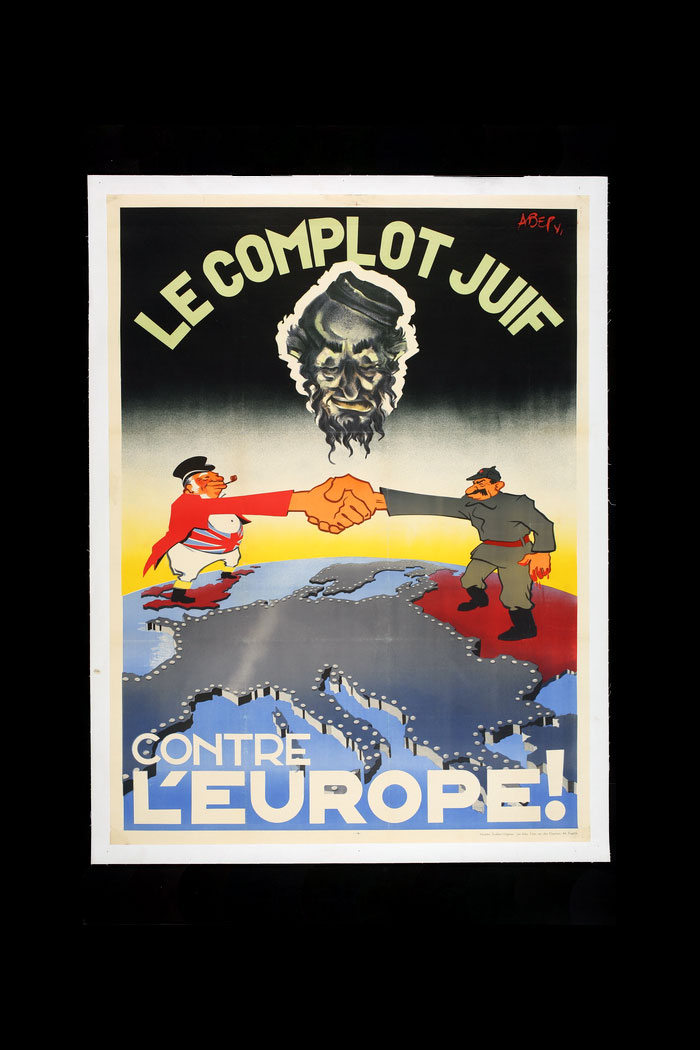The image depicts a vertically oriented political poster with a black background and a white border. The poster features the French title "La Complote Juive Contre l'Europe" at the top, which translates to "The Jewish Conspiracy Against Europe." 

Central to the poster is a detailed map of Europe. Western Europe is colored blue, while Russia and the United Kingdom are marked in red. The poster also showcases a man dressed in a red and white suit with a black top hat, standing on the UK. This man has a distinctive appearance, complete with a tobacco pipe, white pants, and black shoes. He is shaking hands with another man stationed in Russia, who is wearing a grey Soviet-style uniform with a red belt and a hat, and has a mustache and a beard. Notably, this Soviet-uniformed man has his left hand covered in blood, which adds to the sinister implication.

Hovering above them, watching the handshake with a stern gaze, is a man with a full beard and a hat. The handshake between the two central figures appears to symbolize cooperation between the UK and the USSR, suggesting an undesirable alliance. The globe the two men stand on highlights Europe in grey, with blue water providing contrast.

A clean white frame encloses the poster, and a signature is visible in the upper right corner. The bottom of the poster prominently features the phrase "La Complote Juive Contre l'Europe!" with an exclamation point, which underscores the poster's provocative message.